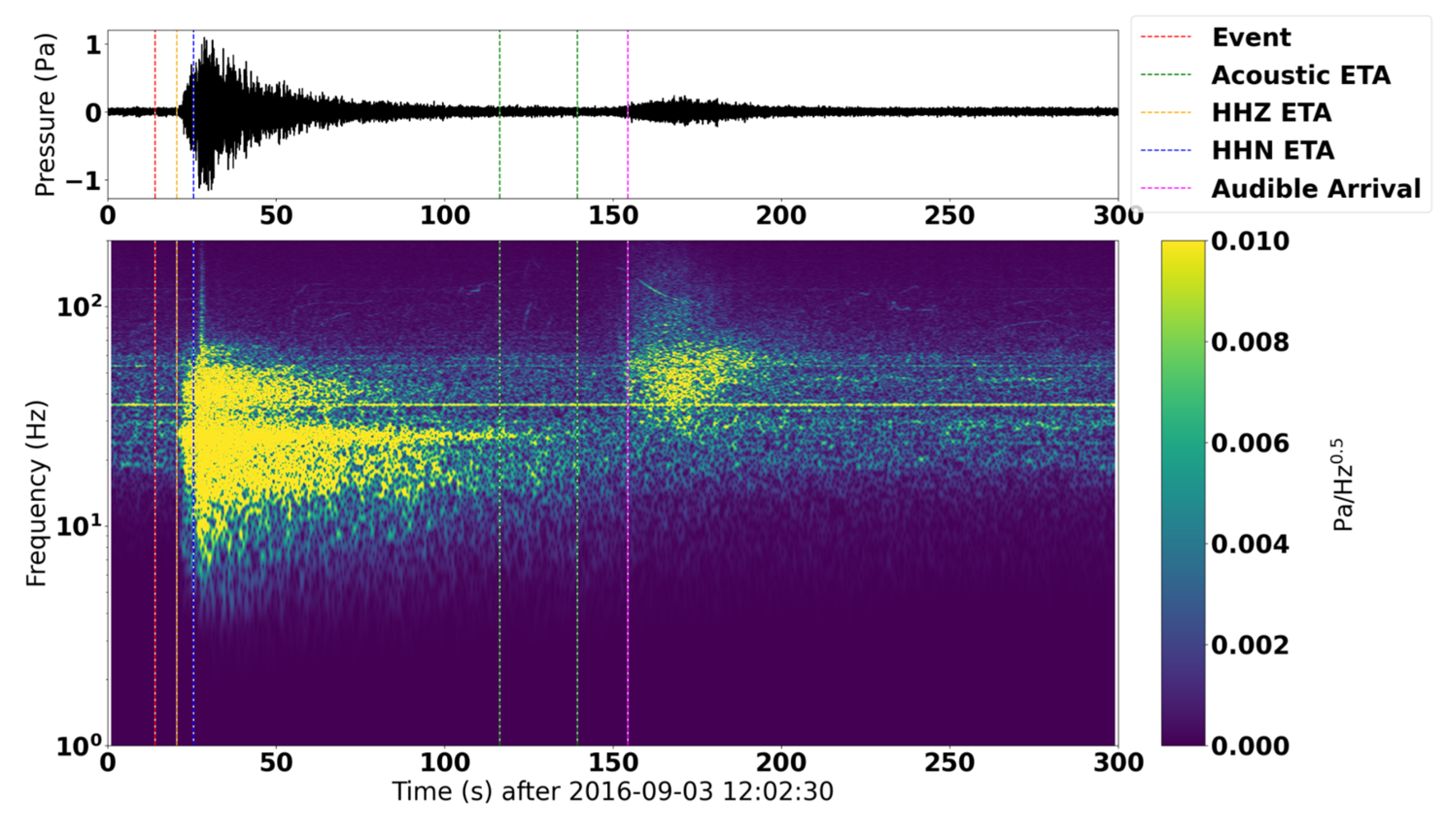The image displays a detailed seismogram graph, split into two sections. The top portion features a black and white graph labeled "Pressure (PA)" on the left, marked with the numbers 1, 0, and -1. Horizontally, it is segmented with intervals of 50 from 0 to 300. At the top right, a legend identifies color-coded lines: red for "Event," green for "Acoustic ETA," yellow for "HHZ ETA," blue for "HHN ETA," and pink for "Audible Arrival."

Below this, a larger graph with a blue background is shown. It is labeled "Frequency (Hz)" on the left, with logarithmic scales indicated as 10^2, 10^1, and 10^0. The bottom axis is marked "Times after 2016-09-03 12:02:30," with intervals from 0 to 300 in steps of 50. To the right, a gradient scale ranges from 0.000 to 0.010, suggesting varying intensities represented by colors transitioning from dark blue to green to yellow. This section visually models frequency data over time, providing a comprehensive view of seismic activity and related acoustic events.